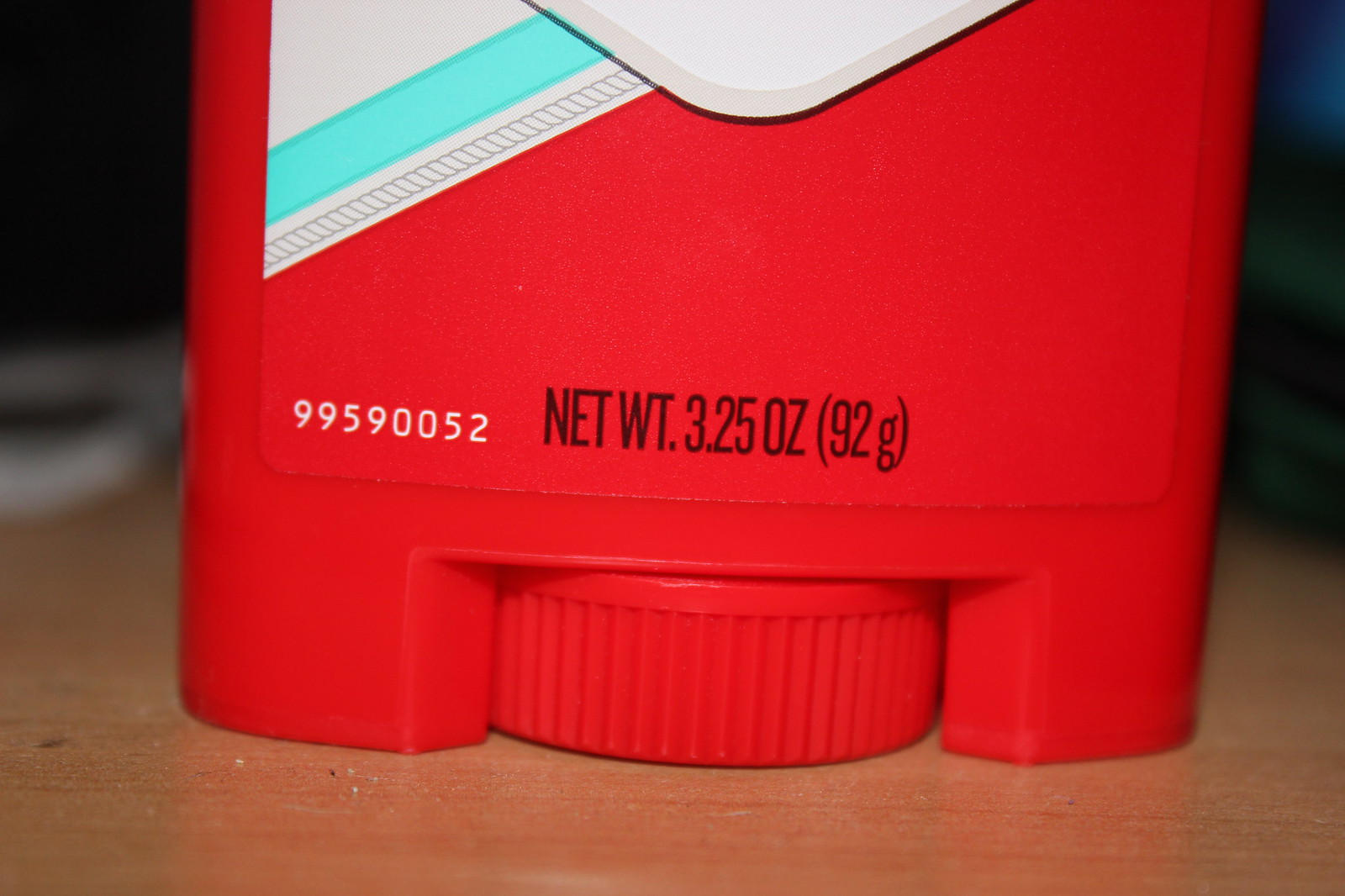A partially visible plastic container, primarily red with accents of white and light blue, is positioned on a very smooth laminate table, which is scattered with dirt, crumbs, and specks of dust. The visible lower half of the container displays black text that reads "Net Weight 3.25 Ounces (92 grams)." Just below this text, there is a red turn dial typically found on antiperspirant deodorant products. The upper half of the container features a white label bordered in black. The overall shape, weight, and design strongly suggest that this is an antiperspirant deodorant.